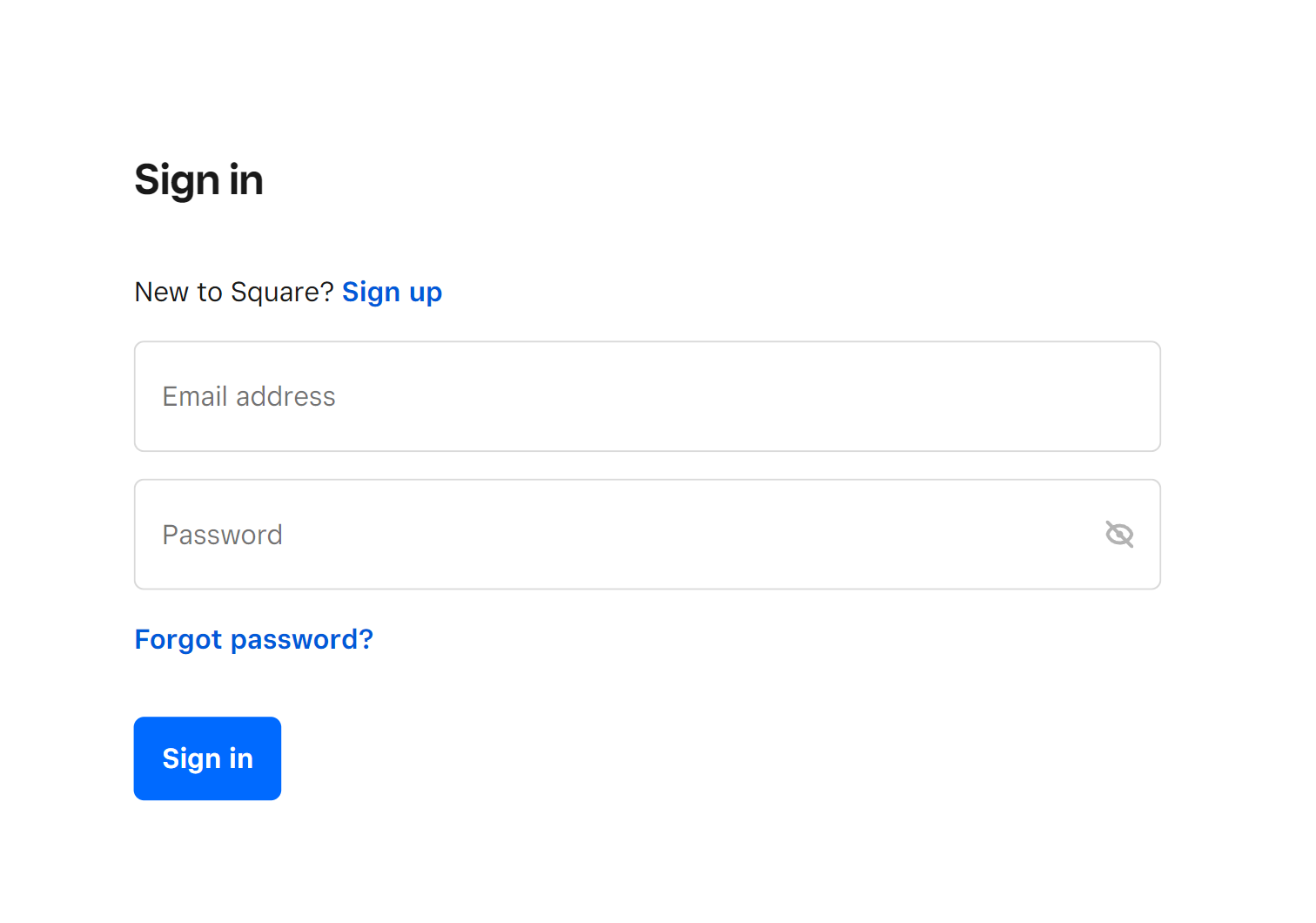The image is a screenshot of a minimalistic login prompt for a service called Square. The background is white, and at the top left corner, bold black text reads "Sign In." Just below, there's some spacing followed by the text "New to Square?" which is posed as a question to new users. Next to this question, "Sign up" is displayed in blue text, indicating a clickable link that presumably directs new users to a registration page.

Further down, two large rectangular input fields are present. The first field is labeled "Email Address," prompting users to enter their email address to log in. The second field, labeled "Password," includes an icon of an eyeball with a strike-through, indicating that the password entered will be obscured for security.

Below these fields, blue text reads "Forgot Password," offering a recovery option for users who cannot remember their password. Finally, at the bottom of the prompt, there is a prominent blue button with white text that says "Sign In," which users would click to submit their login credentials.